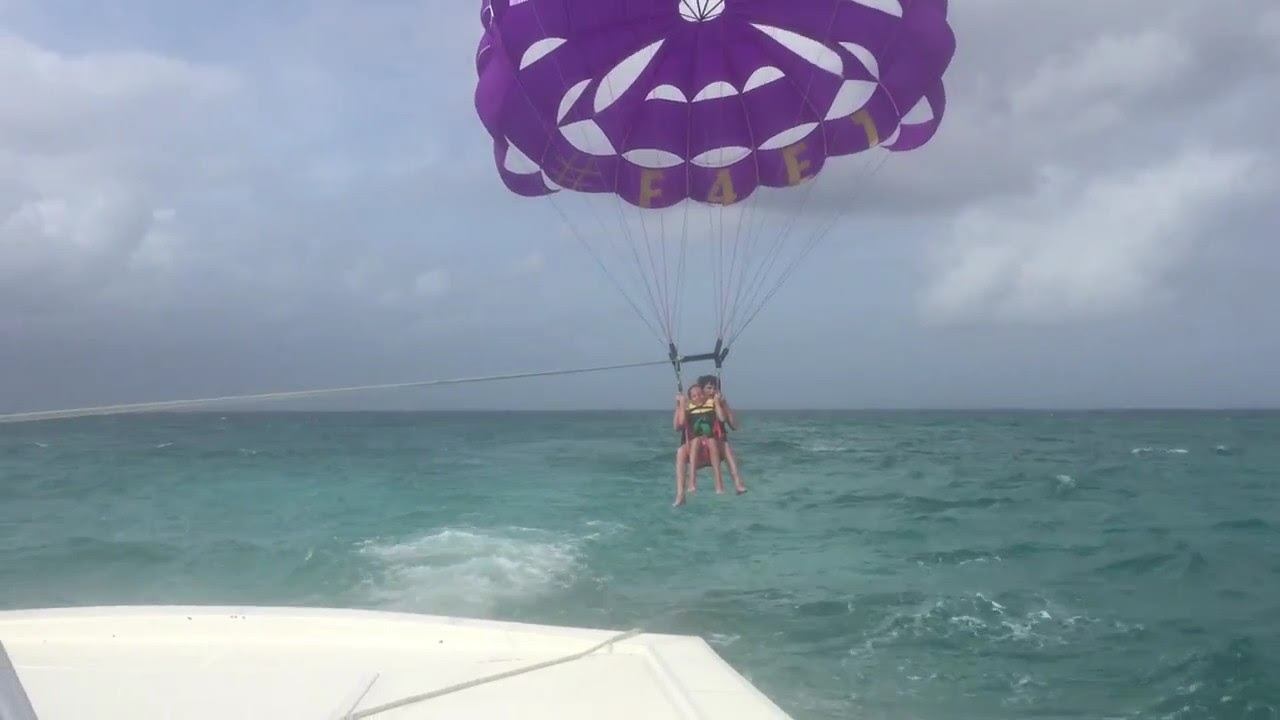In the image, two young individuals, likely teenagers, are parasailing over a greenish-blue ocean. They are suspended in the air by a large parachute that is predominantly purple with white scalloped designs and a white circular spot in the center. The parachute has the hashtag "F4E1" inscribed in pale gold on its edge. Both individuals are wearing life jackets—one appears to be yellow and black. They are seated together in the same harness, with their legs dangling freely. The parasail is tethered to a white boat, which is visible from the rear in the bottom right of the picture, skimming over slightly choppy waves. The sky above is mostly cloudy with large gray clouds, and hints of blue sky peeking through, indicating a possibly overcast or late afternoon setting.